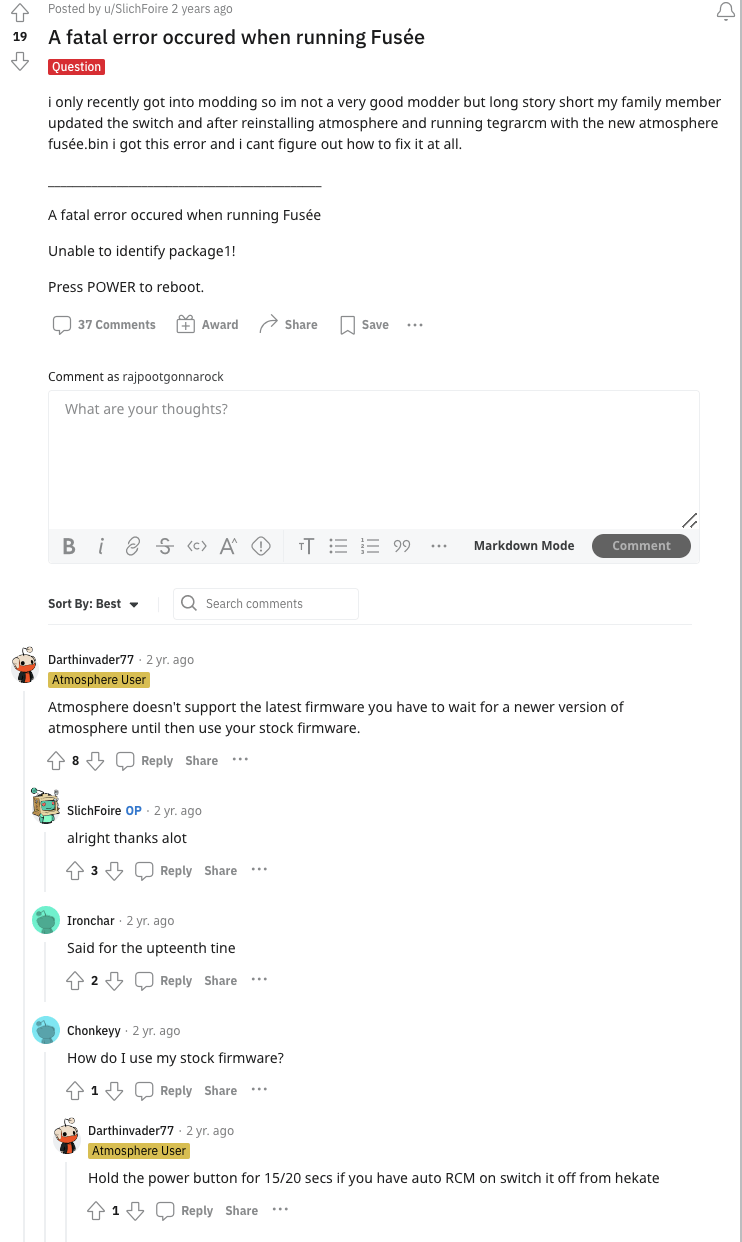Here is a detailed and cleaned-up caption for the described image:

---

The image displays a forum discussion posted by Sledge approximately two years ago, addressing a fatal error encountered while using Fusee with a modded Nintendo Switch running Atmosphere firmware. The error message, highlighted in a red box, reads: "Fatal error occurred when running Fusee. Unable to identify it. Press power to reboot." 

The user explains that after a family member updated the Switch, they began experiencing issues running the modded firmware. Despite being new to modding, they seek assistance from the community to resolve the error. 

Accompanying the post, there are 37 comments from community members. The interface shows options to award, share, and save the post. Users can type their responses in a comment box, enhanced with features such as markdown mode, text formatting options (bold, italics), and bullet points.

At the top of the comment section, a filter tool allows sorting comments by criteria like 'best.' 

Highlighted is a comment by user Darth Invaders from two years ago, advising: "My Atmosphere doesn't support the latest firmware. You have to wait for a new version of Atmosphere until you can use your stock firmware." 

A follow-up response acknowledges the advice, and another user, Chunky, inquires about using their stock firmware. Darth Invaders directs them to hold the power button for 15 to 20 seconds if auto RCM is enabled on the Switch. 

The forum's background is a clean white, facilitating easy readability of the discussion.

---